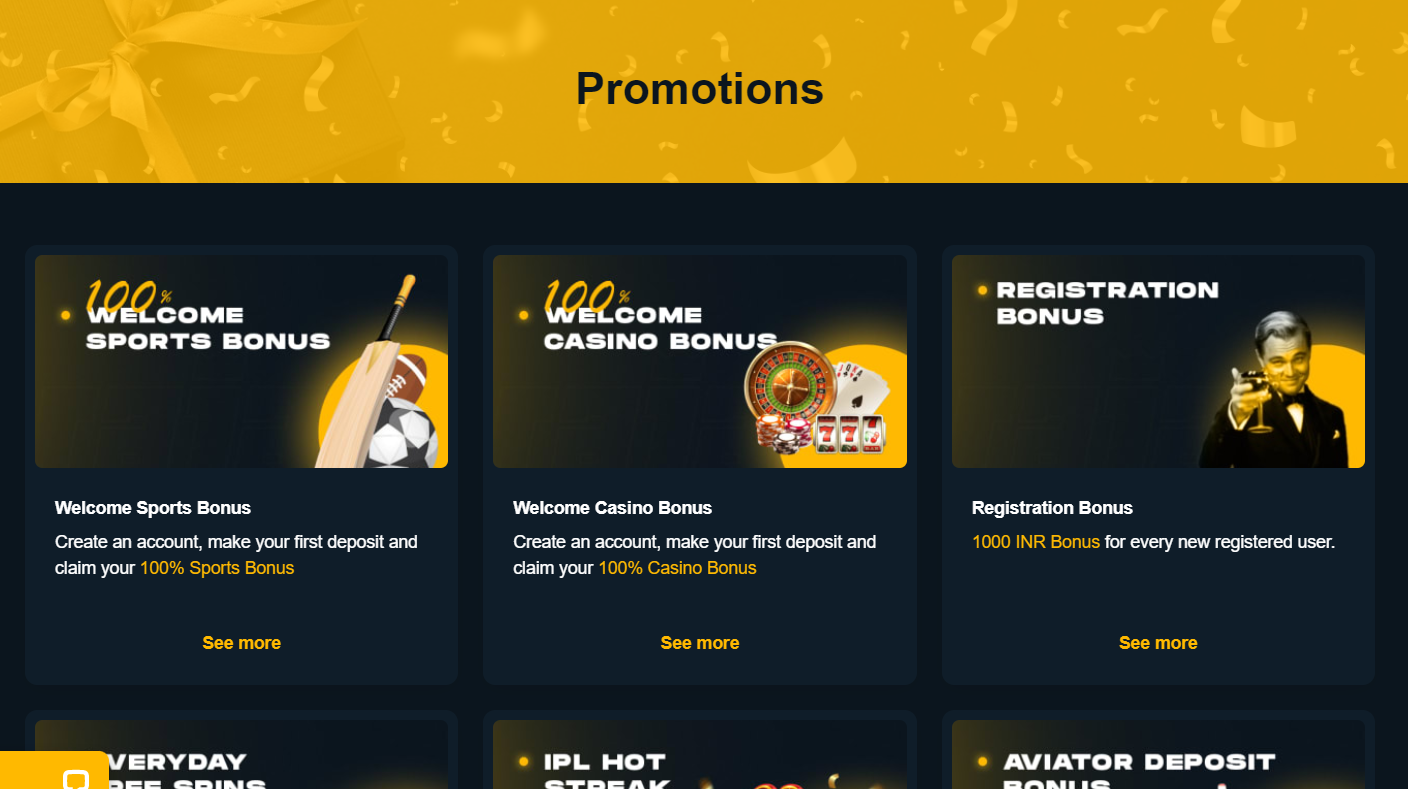The image displays a promotion for a sports and casino bonus registration. At the top of the image, there's a prominent yellow bar with the text "Yellow" on it. Below that, several promotional messages and instructions are vividly displayed. 

A section labeled "Texas Promotions" is followed by the text "Welcome Sports Bonus." The instructions detail how to create an account, make the first deposit, and claim a 100% sports bonus. Additional messages encourage users to "See More" for everyday promotions and include details about the "Welcome Casino Bonus," which offers a 100% casino bonus upon creating an account and making a first deposit.

Another segment highlights the "Registration Bonus," offering a 1000 INR bonus for every new registered user. A person is shown holding up a cocktail, emphasizing the celebratory mood of the promotions. 

In a yellow circle, there's a note about the "Aviator Deposit Bonus" amidst a dark background, adding contrast and drawing more attention to the promotional offers. The bottom of the image features a sequence of six squares, possibly representing steps or additional offers.

Overall, the background is dark, which makes the bright yellow accents and promotional messages stand out prominently.